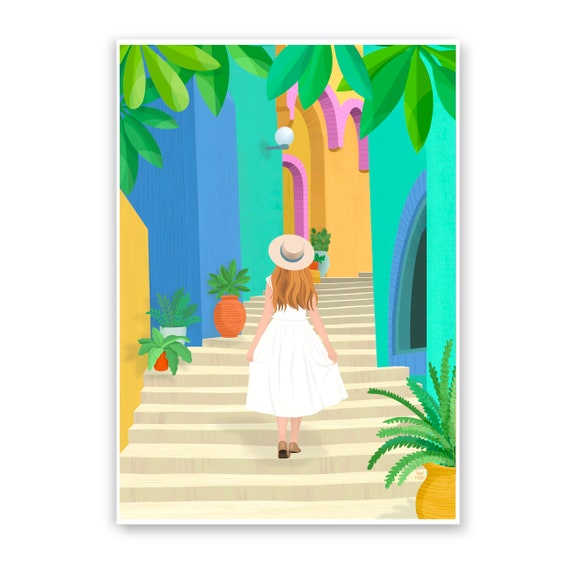The image showcases a meticulously detailed, framed artwork with a white border and drop shadow. The central focus is a young girl with long blonde hair cascading to the mid-lower part of her back, wearing a white dress and brown shoes. She is depicted ascending tan-colored stairs. Adorning her head is a beige hat with a green ribbon. The setting features a vibrant array of colorful buildings in shades of teal, blue, yellow, and magenta. Additionally, there are potted plants situated on various steps and green leaves hanging from the top of the image, adding to the lively atmosphere of the scene.